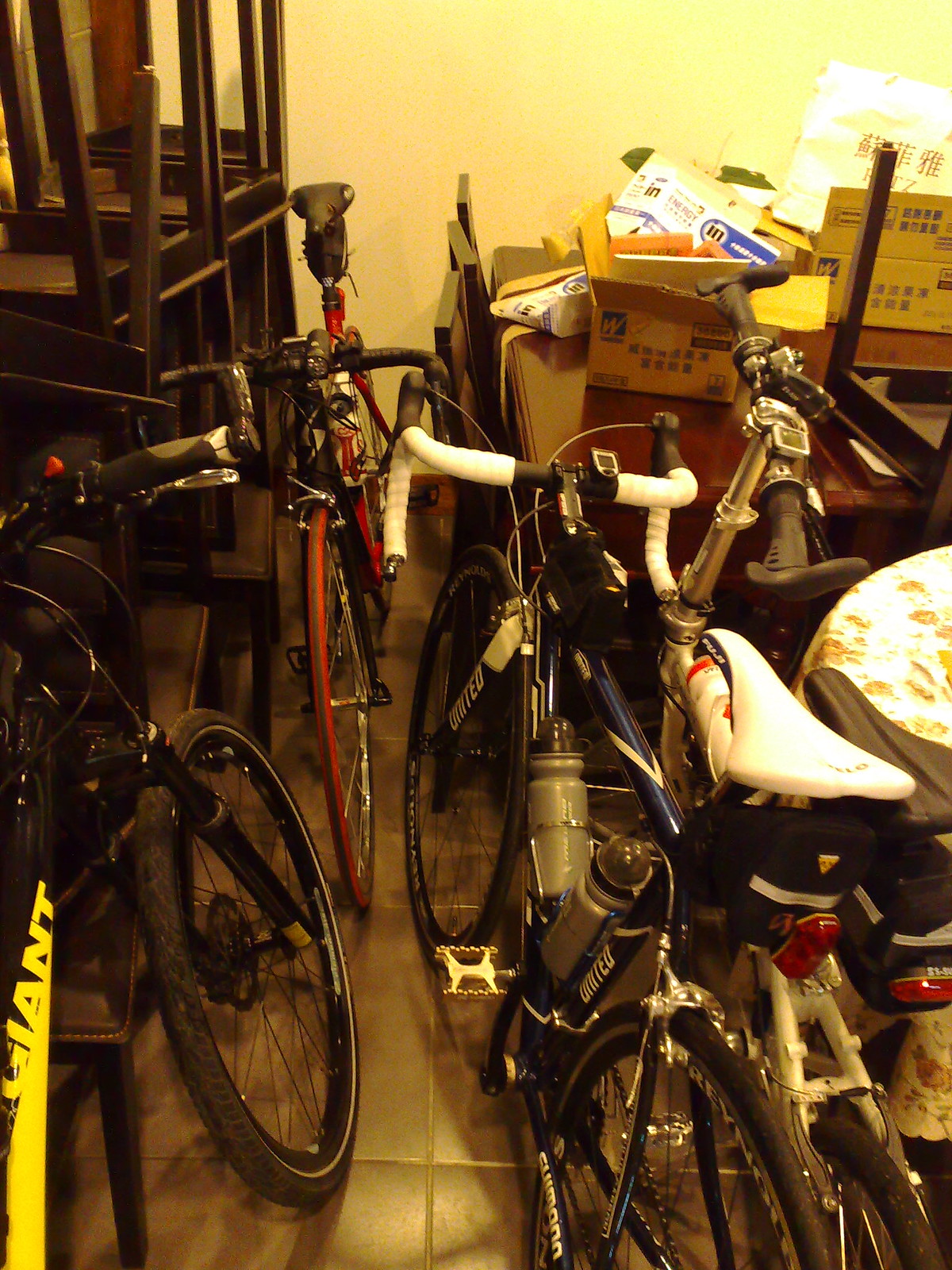The photograph captures a very cluttered room that resembles a messy garage or storeroom, characterized by its yellow wall in the background and large dark tiles separated by gray grout on the floor. In the left-hand side of the image, there are dark brown wooden chairs stacked in pairs with one chair flipped upside down on top of another, legs pointing upward. Leaning against these chairs are two bicycles: a red one and a black one. Dominating the center of the scene is another racing bicycle with distinct curved white handlebars designed for aerodynamic positioning, a gray and black water bottle attached, and a white seat. Further to the right, the clutter continues with more chairs and various pieces of furniture stacked up to about halfway to the ceiling, including what appears to be a matching wooden table beneath the piled-up chairs. In addition to this, the image reveals four bikes: a prominently featured racing bike with thin reddish wheels and a black seat, another racing bike in the background, and a black bike with yellow "Giant" lettering—likely a mountain bike—facing a different direction. Scattered amidst the chaos are boxes filling the space, adding to the sense of disarray.